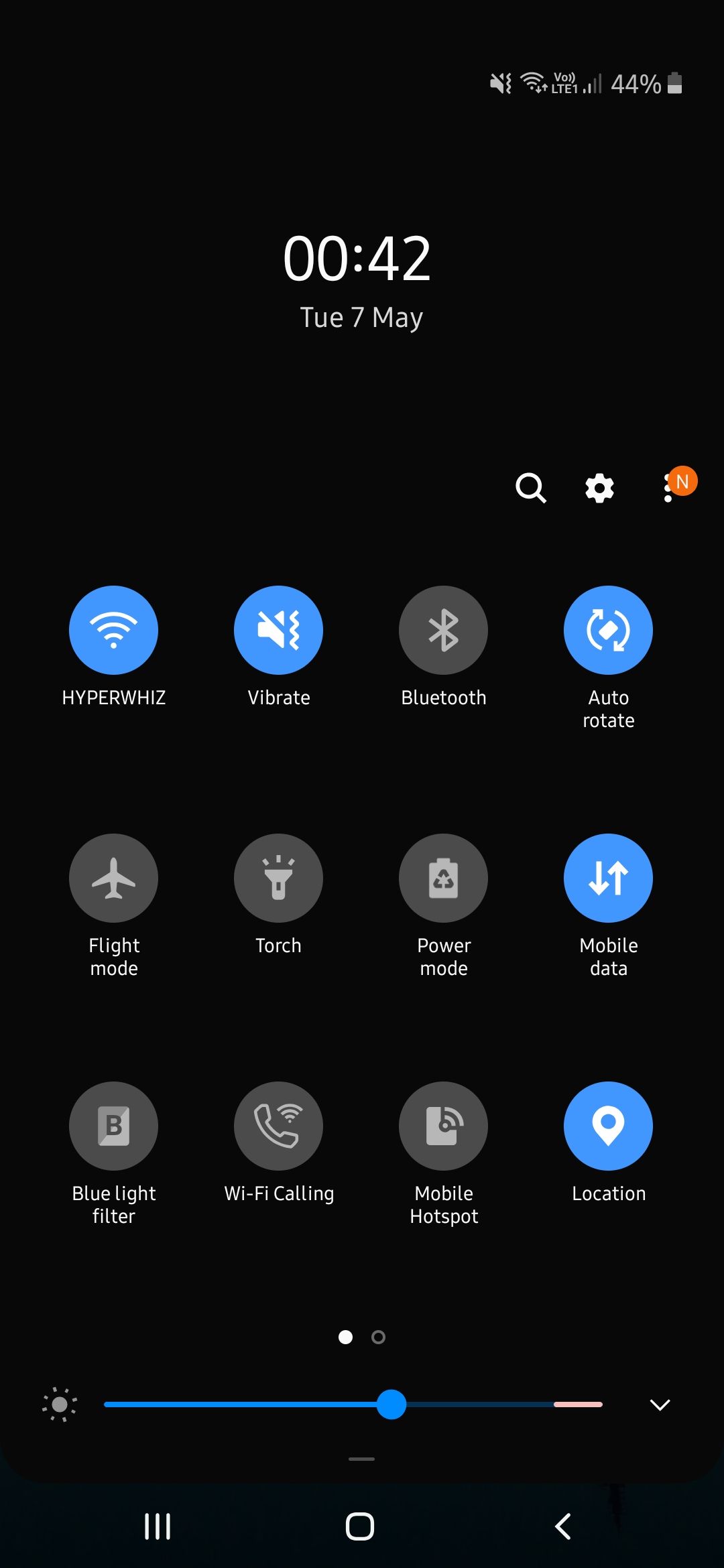The image is a mobile screenshot showcasing a jet black background with various icons and text. In the top right corner, it displays icons including the battery level at 44%. Centered at the top is the time, "00:42" and the date, "TUE 7 May". To the right, there is a magnifying glass (search icon), a settings icon, three vertical white dots, and a circular icon with the letter "N".

The main menu features 12 icons with corresponding text. The top row displays icons for Wi-Fi, sound settings, Bluetooth, and auto-rotate settings. Wi-Fi, sound, and auto-rotate settings are highlighted in blue with white icons, indicating they are enabled. Bluetooth is gray with a white icon, indicating it is disabled. 

The second row contains icons and text for flight mode, torch, power mode, and mobile data. The mobile data button is highlighted in blue, signaling it is active. 

The third row has icons for blue light filter, Wi-Fi calling, mobile hotspot, and location. The location button is highlighted in blue, showing it is enabled.

At the bottom of the screenshot, there is a brightness slider, colored blue with a blue circle located slightly past the halfway mark to the right. Below the slider are three navigation icons.